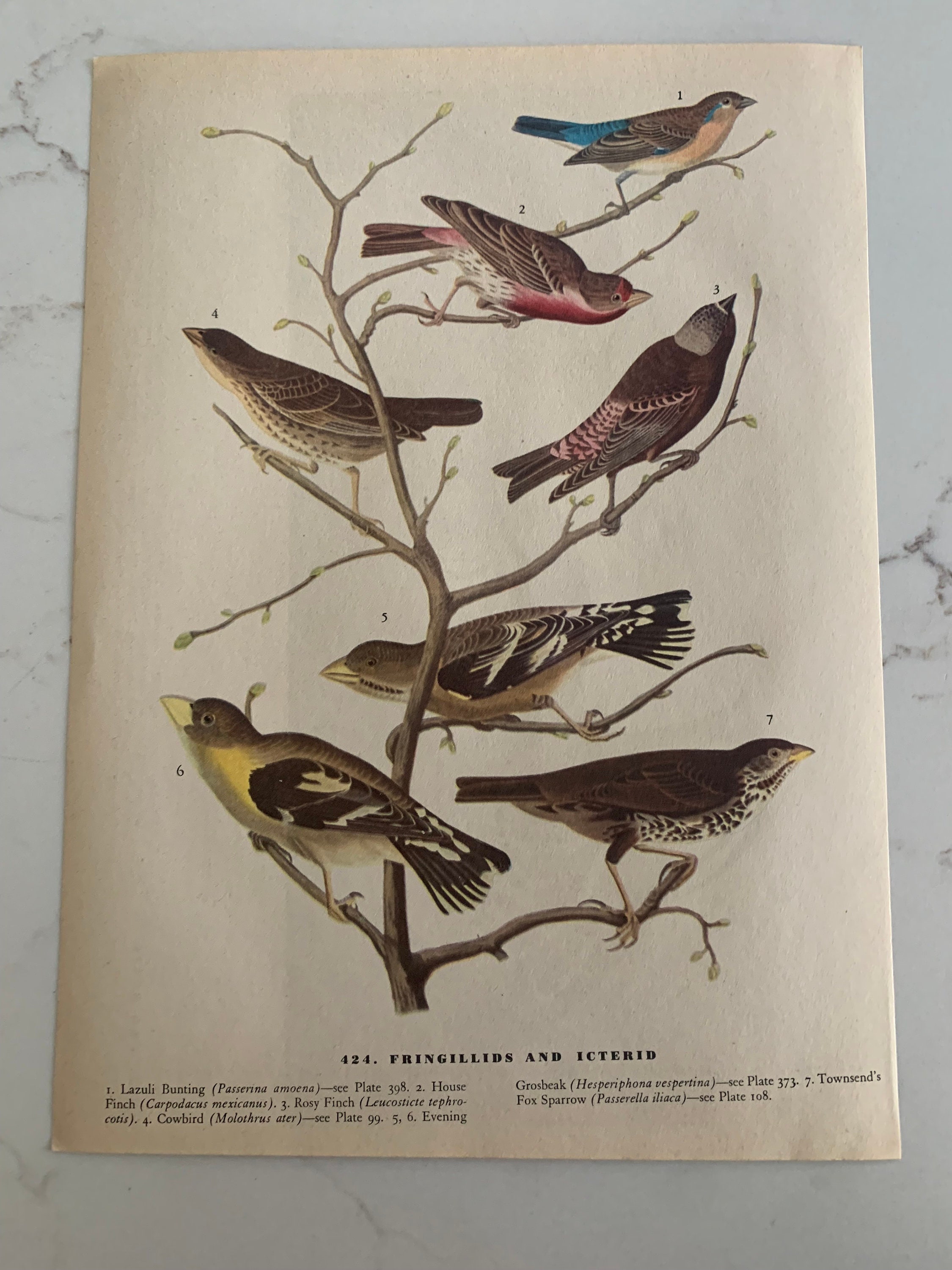This image is an excerpt from a book or encyclopedia page focused on birds, likely phryngolids and ichthyorids, as indicated by the fine print at the bottom that reads "424 phryngolids and ichtorid." The paper, rectangular and resembling a piece of a textbook or notebook, lies on what appears to be a marble counter or table. Central to the illustration is a tree branch with various smaller branches extending horizontally, each supporting one of seven distinct birds. The avian figures, which appear meticulously drawn or painted, include a variety of colors: one bird stands out with vibrant yellow, another with striking blue, two with red highlights, and the remaining three predominantly brownish with differing decorative patterns. These birds' unique characteristics are underscored by the numbered annotations and Latin names beneath them, akin to a field guide layout. Some birds gaze left while others look right, contributing to the lifelike scene. The detailed and intricate artwork on the page, complemented by a mix of textual and scientific notation, makes it a rich visual document likely intended for educational purposes.